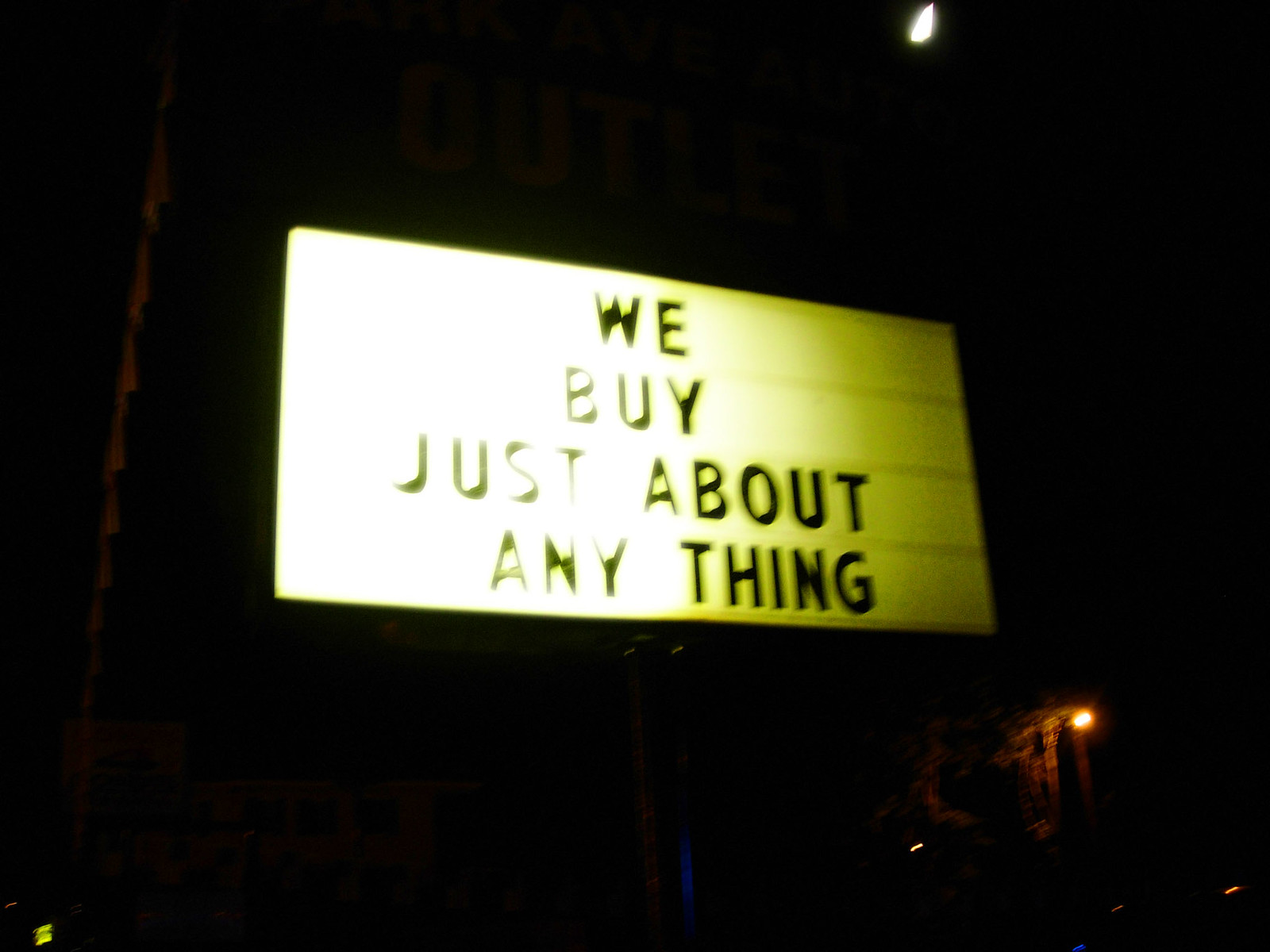The image is a slightly rectangular frame with a predominantly black background, evocative of a nighttime outdoor setting. In the lower right corner, the faint outline of a building can be discerned, subtly illuminated by an exterior light that casts a dim, orange hue across the area. The focal point of the image is a sign located on the left side. The sign features a bright white background that gradually fades into a yellowish color. It is the type of sign used for placing interchangeable letters. Centered on the sign in four rows of black letters is the message: "We Buy Just About Anything."